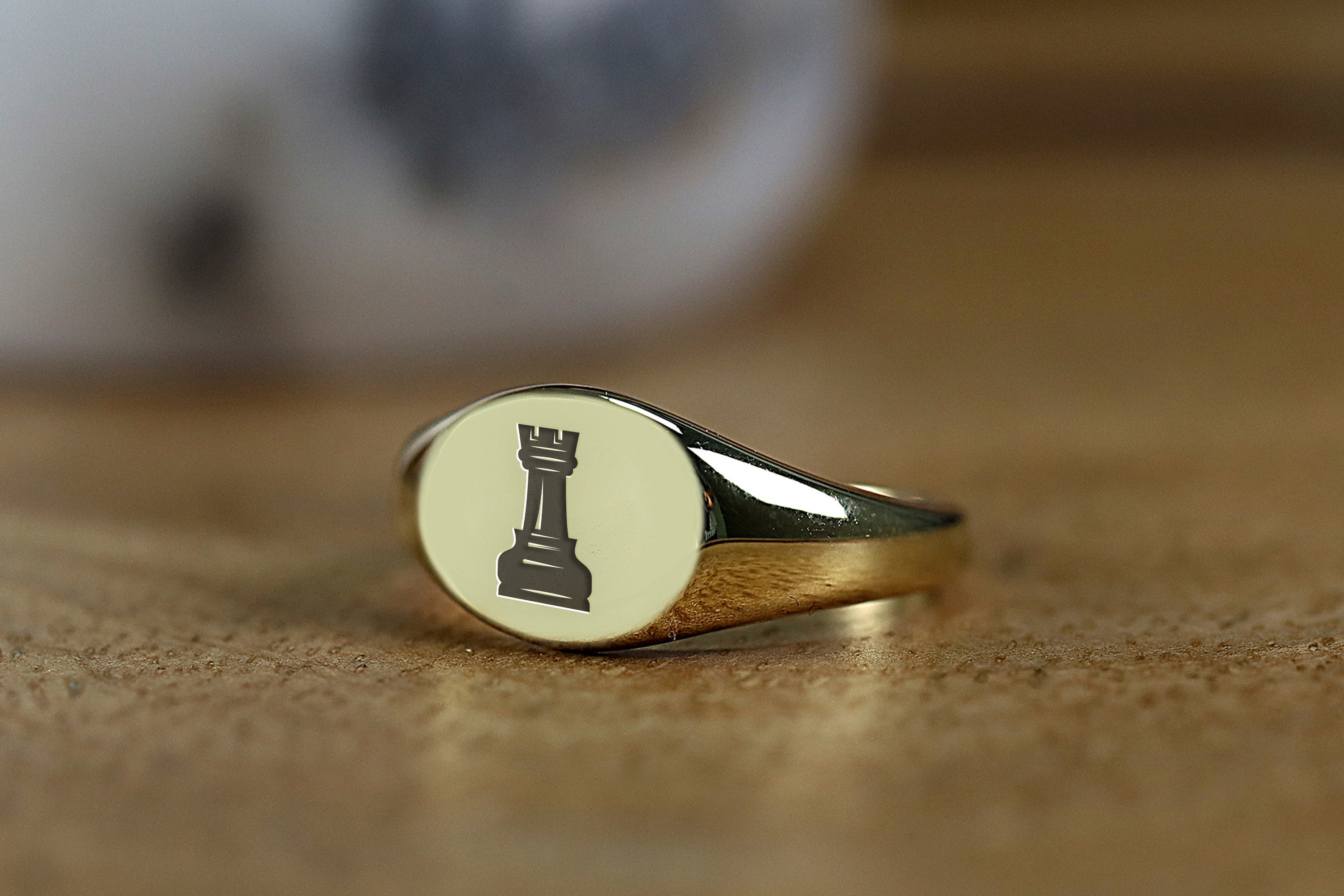The image displays a sterling silver ring resting on a brown wooden tabletop. The ring's face is flat and smooth, adorned with a pale beige-yellowish hue. Prominently featured on this flat surface is a detailed illustration of a dark grey queen chess piece. Notably, the metal encircling the pale face of the ring is highly reflective, capturing a faint reflection of the person taking the picture. The background is blurred, with an indeterminate large white object, possibly a pot or vase with blackish-blue markings, vaguely visible behind the ring. The face of the ring is slightly angled away from the camera.